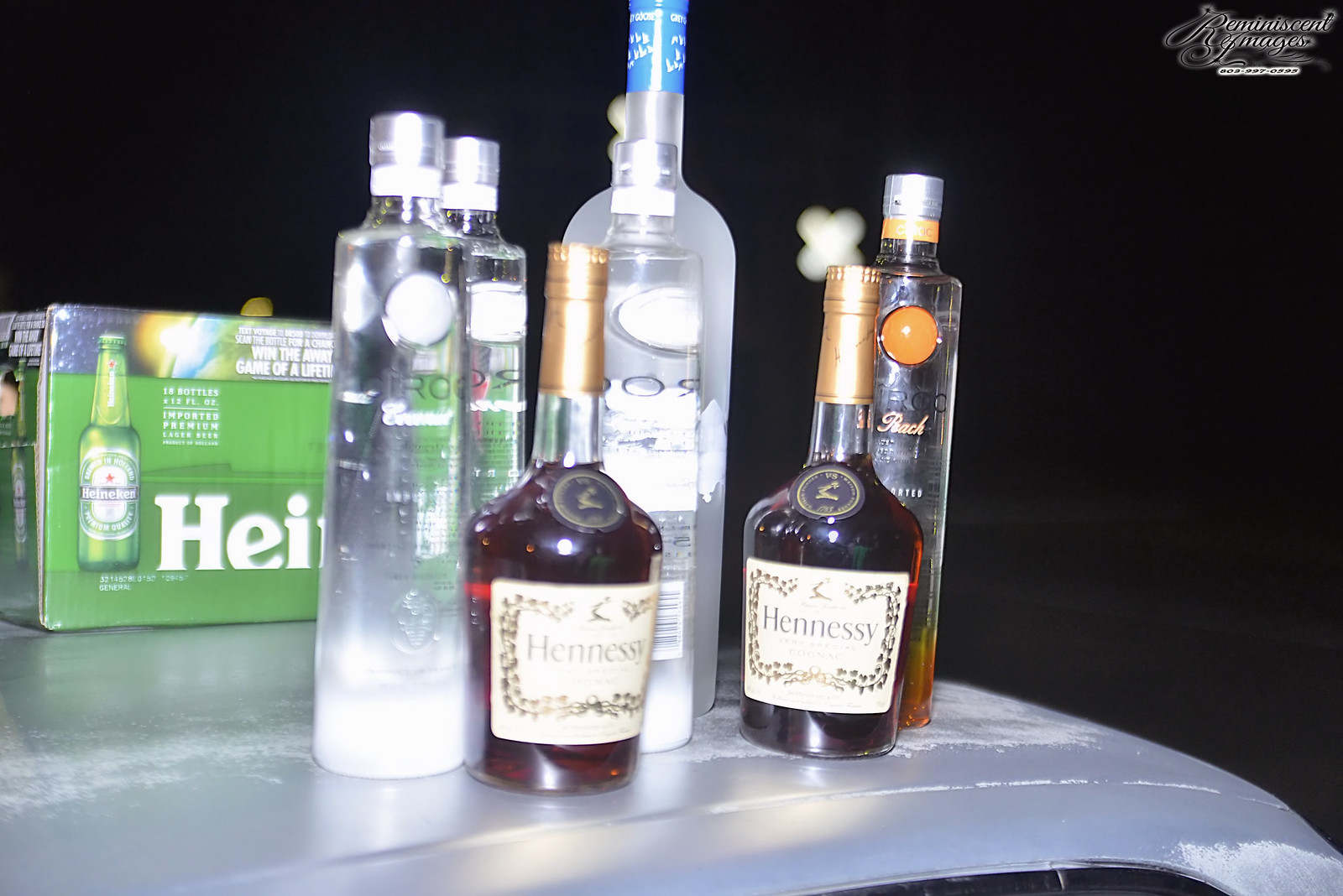The photograph captures a collection of liquor bottles arranged on a curved metal surface, possibly the roof of a car, set against a dark, almost black background indicative of nighttime. Central to the image are two Hennessy bottles with gold caps, the amber liquid inside clearly visible. Flanking these bottles to the left are two slender bottles holding a clear liquid, potentially Ciroc vodka, with one likely being peach-flavored. Positioned in the middle is a bottle featuring a rounded top and blue cap. On the far right is a bottle with a silver cap, containing a liquid that transitions from brown at the bottom to clearer towards the top, suggested to be Grey Goose vodka. Behind all the bottles, there's an 18-pack case of Heineken beer. Additionally, in the top right corner of the image, there is a partially visible sign or card with an 803 area code, labeled as "Re-Reminiscent Images." Some chrome detailing, possibly from the car, can be faintly seen along with minor scuff marks.